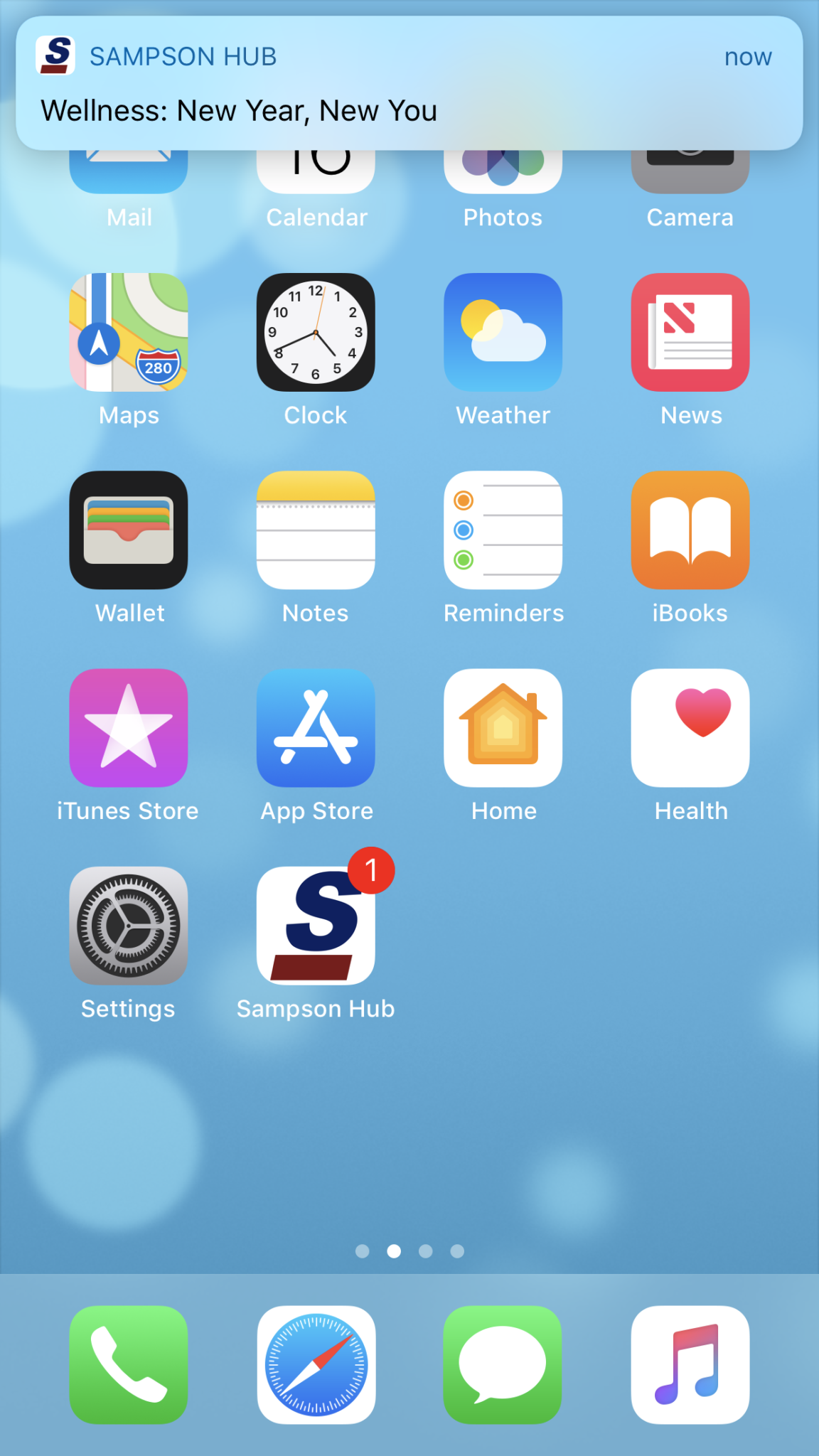The image depicts a smartphone home screen featuring various application icons arranged in a grid layout with four icons per row. At the top, there are widgets for "Samsung Hub," "Wellness," and a New Year-themed banner. The background is primarily blue, adorned with several circles. 

Here are the app icons displayed, along with their descriptions:

1. **Samsung Hub**: Represented by an 'S' with a line through it, located in the top right corner inside a red circle.
2. **Wellness**: Positioned at the top.
3. **New Year, New Year**: Possibly a widget for the festive season or an event countdown.
4. **Texas is Now**: Indicated in blue, possibly referring to a location-specific app or event.
5. **Calendar**: Standard calendar icon.
6. **Photos**: Standard photo gallery icon.
7. **Camera**: Standard camera icon.
8. **Maps**: Standard maps icon.
9. **Clock**: Standard clock icon.
10. **Weather**: Standard weather app icon.
11. **News**: Standard news app icon.
12. **Wallet**: Displayed with a wallet icon.
13. **Notes**: Represented by a notepad icon.
14. **Reminders**: Standard reminders icon.
15. **iBooks**: Standard iBooks icon.
16. **Star**: Generic star icon.
17. **iTunes Store**: Standard iTunes Store icon.
18. **App Store**: Standard App Store icon.
19. **Home**: An orange icon with a white house.
20. **White Skirt with a Red Heart**: Possibly an app icon or folder with a clothing-related image.
21. **Settings**: Gray gear icon.
22. **Green Phone**: Standard phone app icon, on a green square background.
23. **Compass**: Standard compass icon.
24. **White Square with a Music Note**: Possibly a music-related app, with a blue background.

The bottom row has four circle icons, which might be indicators or additional widgets. The home screen effectively showcases a typical smartphone layout with organized rows of commonly used applications.